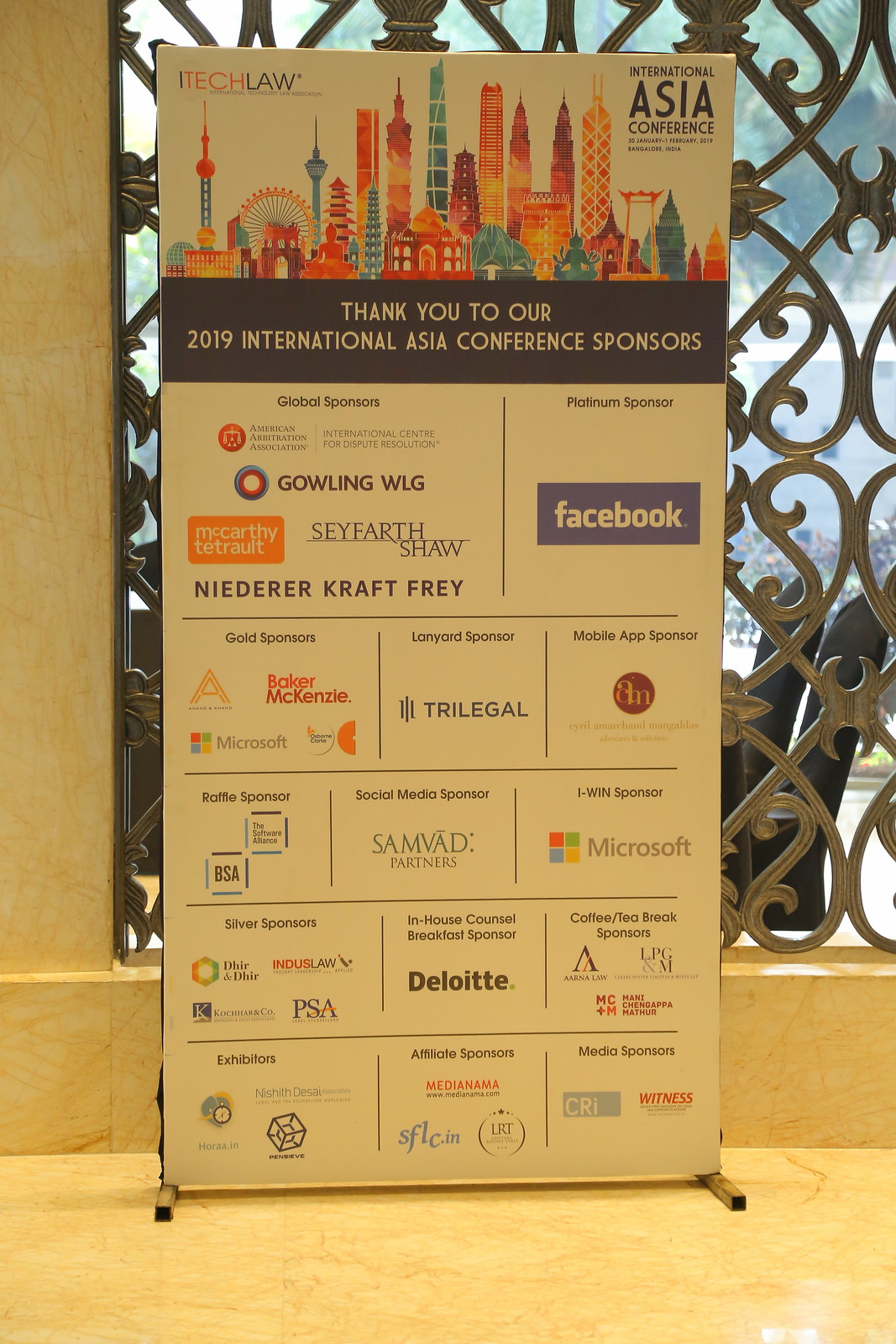This image depicts a large, stand-up banner prominently displayed in what appears to be the luxurious marble-floored lobby of an event venue. The marble walls and floor add to the high-end setting, with their shiny, yellowish surfaces accented by intricate swirls. The banner itself, primarily white and mounted on a silver stand, serves as a significant centerpiece within the opulent surroundings.

At the top of the banner, bold text announces "iTech Law International Asia Conference," accompanied by a vibrant illustration of skyscrapers and towers creating a colorful city skyline on the upper right side, possibly representing an Asian metropolis. Directly beneath, a black-bordered section reads, "Thank you to our 2019 International Asia Conference sponsors," leading into a detailed list of various sponsor categories.

Among the numerous sponsors acknowledged are global sponsors like Gowling WLG, Seyfarth Shaw, McCarthy Tetrault, and Niederer Kraft Frey. Platinum sponsors include major companies such as Facebook, while Microsoft is noted among other contributors. Additionally, there are specific designations for different types of support, such as a mobile app sponsor (Cyril Amarchand Mangaldas), gold lanyard sponsor, raffle sponsor, social media sponsor, silver sponsors, in-house counsel breakfast sponsor, coffee/tea break sponsors, exhibitors, affiliate sponsors, and media sponsors. The range of companies listed spans well-known global entities to smaller, perhaps less recognizable names, illustrating a diverse and extensive network of support for the event.  

The surroundings of the banner include a metal grate and what appears to be an outdoor view, further adding to the sophisticated atmosphere of the venue.